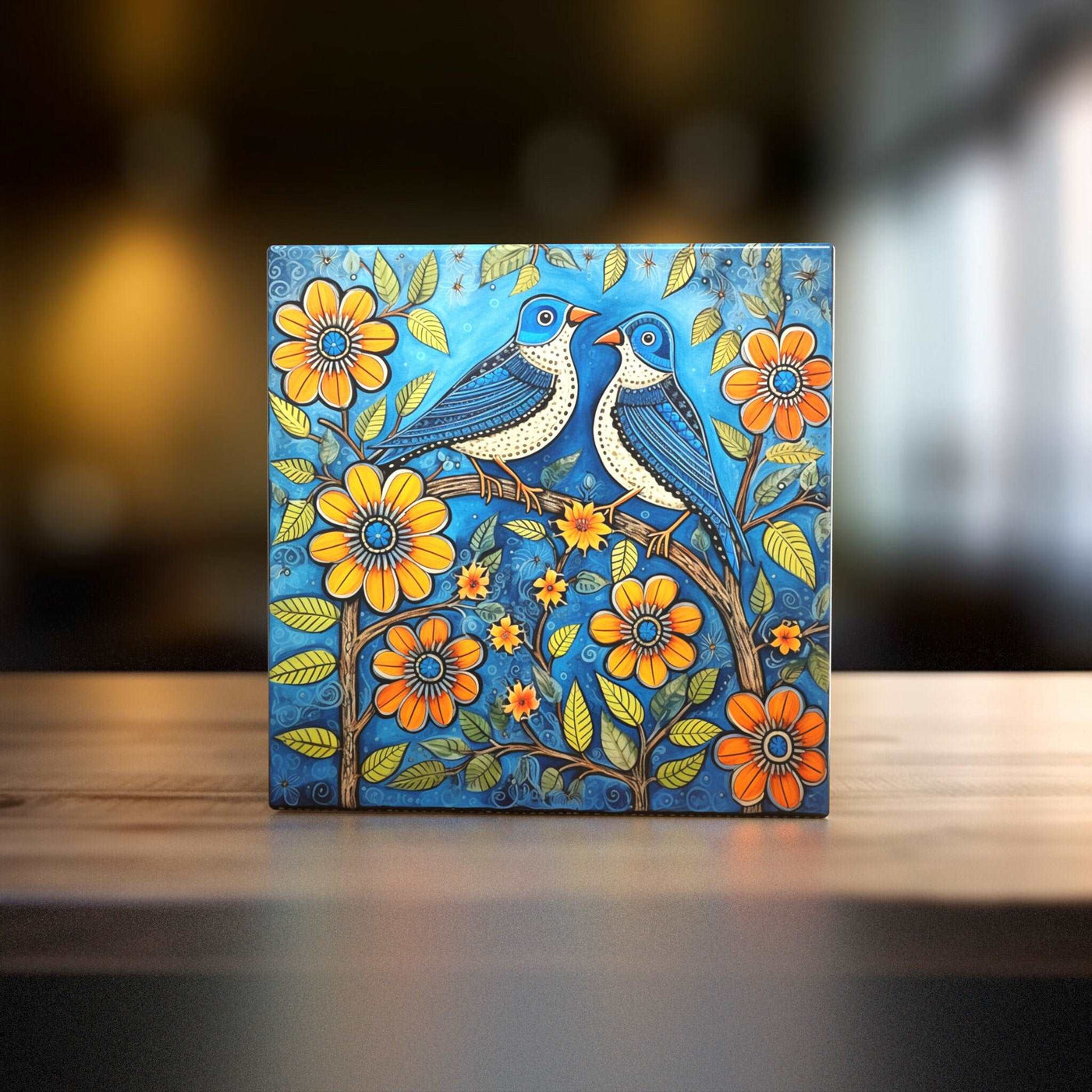The image features a square canvas or tile with a vivid blue background, centrally placed on a wooden table. The artwork depicts two blue birds with orange beaks and speckled white fronts, perched on a horizontal tree branch, facing each other. Surrounding the birds are an abundance of flowers and leaves; six large flowers in shades of yellow and orange, along with several smaller ones and scattered greenery. The photograph blurs everything outside the immediate focus on the canvas. To the left, a yellow-orange light source illuminates the scene, potentially creating a warm glow, while on the right, a softer white light, likely from a window, provides additional background contrast. The composition of the scene includes no text or numbers, emphasizing the natural and colorful elements of the artwork.